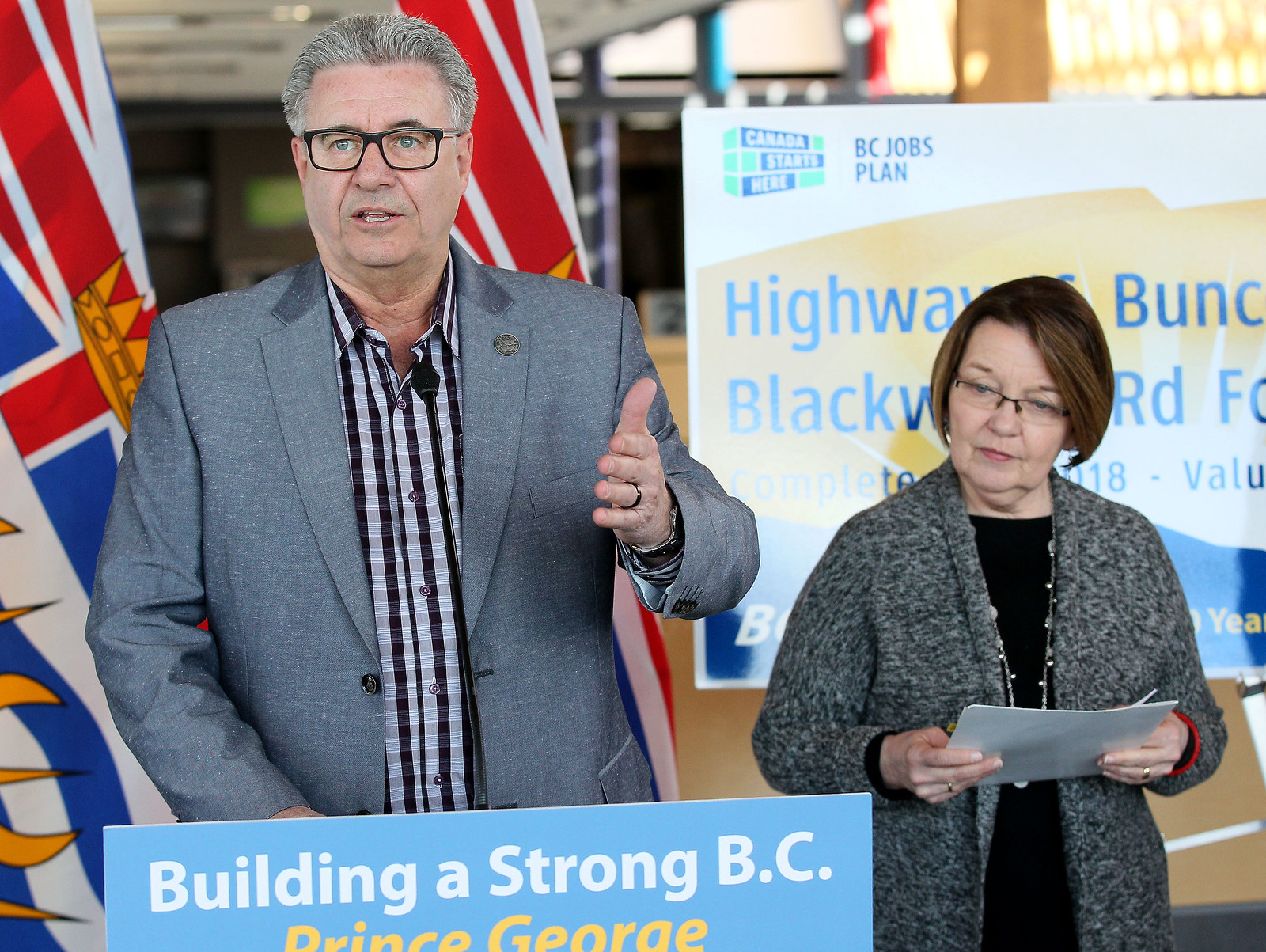In this image, a political event or campaign is underway, featuring a man and a woman prominently. The man, likely a politician, is delivering a speech from behind a podium with a blue background that reads "Building a Strong B.C." in white text and "Prince George" in yellow beneath it. He is dressed in a gray suit jacket, a gray and black striped dress shirt, and black-framed glasses, and has gray hair. To his left stands a woman with brown hair, wearing a gray long sweater over a black shirt, a long necklace, and glasses. She holds some papers, possibly preparing to read from them. Behind them are several flags in red, white, and blue, although their specific designs are not fully visible. The setting appears to be outdoors, hinted by the sunlight to the right, though they seem to be under some sort of covering. A secondary sign in the background reads "Canada Starts Here, BC Jobs Plan," partially obscured by the woman. The edges of the sign contain partly visible text including "Highway," "Road," and "Complete," along with some numbers and the word "value," with other portions cut off.